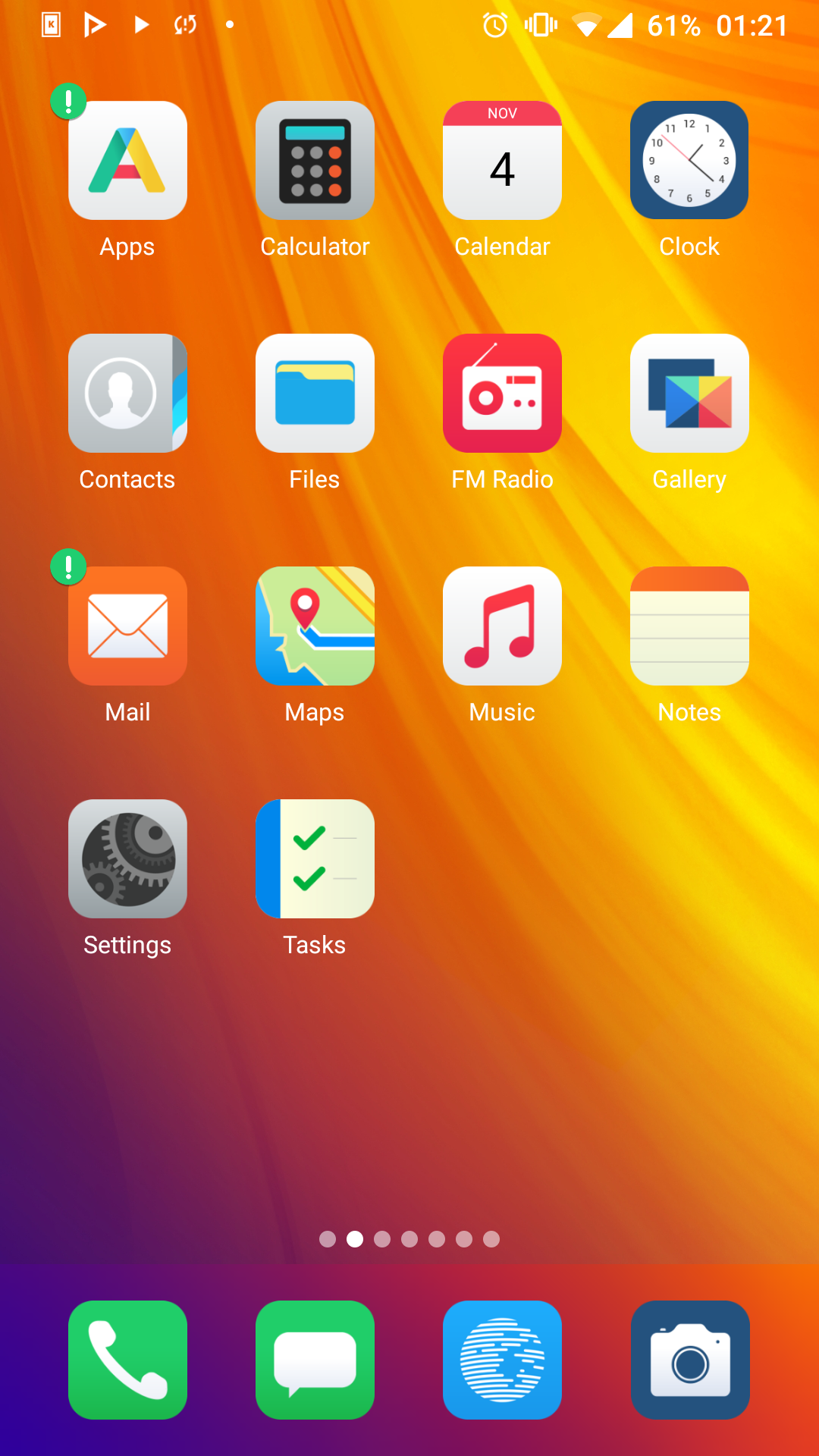A detailed screenshot showcases the second of seven home screens on a smartphone, framed by the devices' standard status and navigation menus. At the top, the status bar displays the current time, battery level, signal strength, and several app notifications, including a system alert. The bottom navigation bar features essential favorite icons for phone calls, text messages, internet browsing, and the camera app. The home screen's colorful gradient background, blending hues of yellow, orange, and purple, accentuates the neatly arranged app icons. The applications visible on this page include Calculator, Calendar, Clock, Contacts, Files, FM Radio, Gallery, Mail, Maps, Music, Notes, Settings, and Tasks.